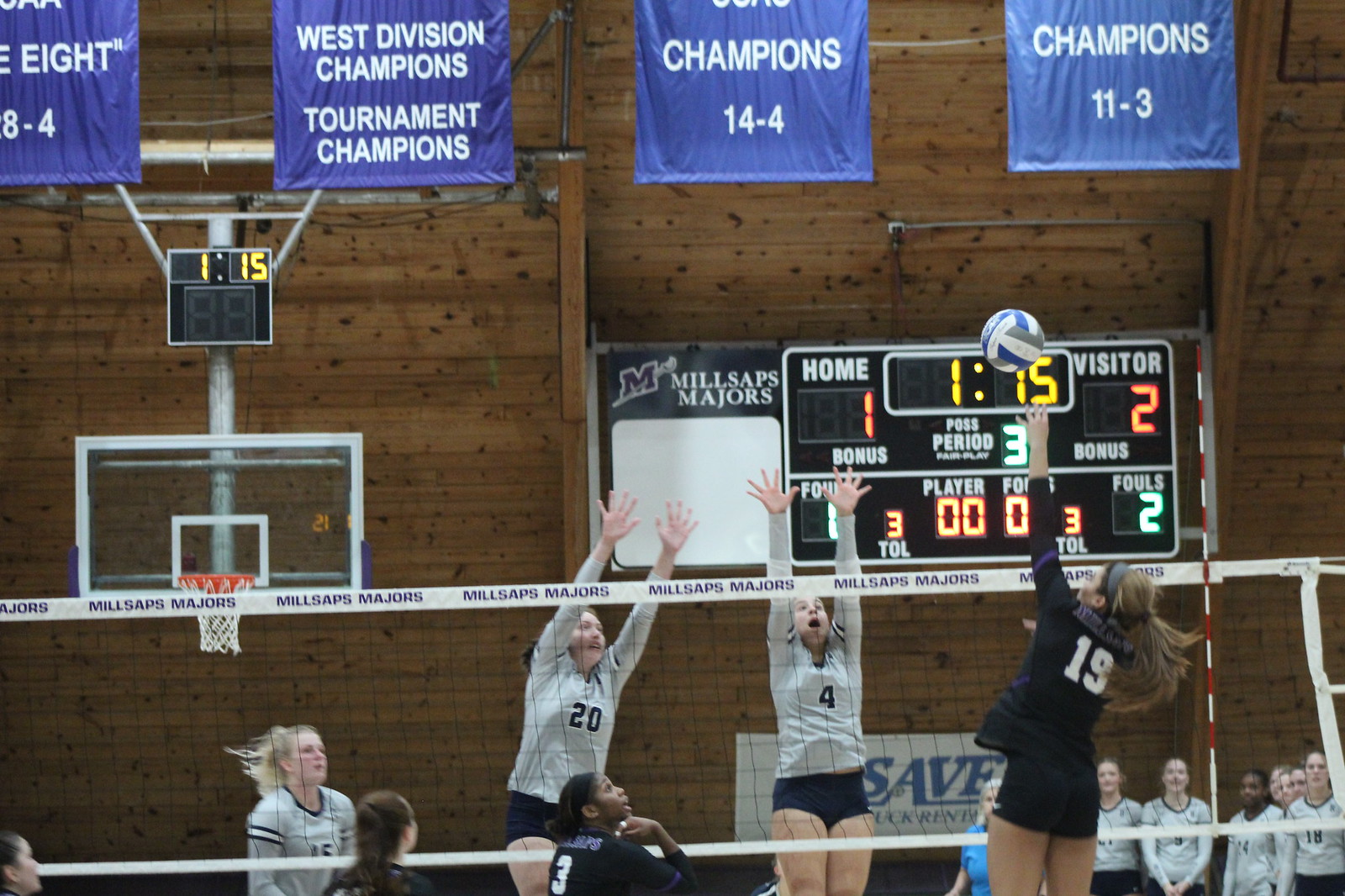In a high-ceilinged wooden gymnasium, a women's volleyball game unfolds beneath a scoreboard reading "Home 1, Visitors 2" with 1:15 remaining in the third period. Blue banners, declaring titles like "West Division Champions" and "Champions 14-4," adorn the walls above the wooden-paneling. Below them, "Millsaps Majors" is prominently displayed behind a basketball goal. On the court, three players in gray tops from one team, numbers 4, 15, and 20, are set to block as number 19 from the opposing team, donning dark blue, leaps to spike the ball. Her dark hair is tied back in a long ponytail. Two teammates, including number 3, an African-American girl, watch intently, poised to support the play. The dynamic scene captures the intensity and focus of the athletes in mid-game.